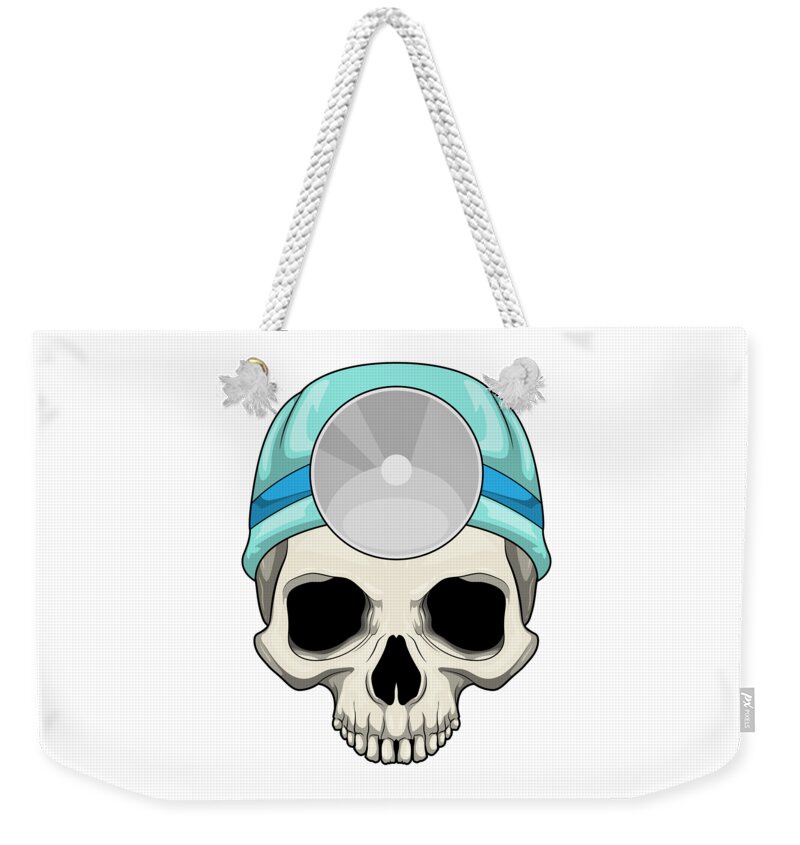The image features a white, rectangular textile bag with a textured pattern and a pair of thick, braided white rope handles attached through small punch-outs near the top left and right edges. On the bag's lower right corner, there is a small, unreadable label that sticks out slightly, reminiscent of a distinctive tag on jeans. The central illustration on the bag depicts a human skull without the lower jawbone, characterized by large, black, sunken eyes and a black nose cavity. Atop the skull sits an aqua blue, skin-tight cap adorned with a bright blue stripe and another stripe of aqua blue. Centered on the forehead of the skull is a classic, silver circular object, often associated with doctors' headwear. The background of the image is entirely white, showcasing the bag.